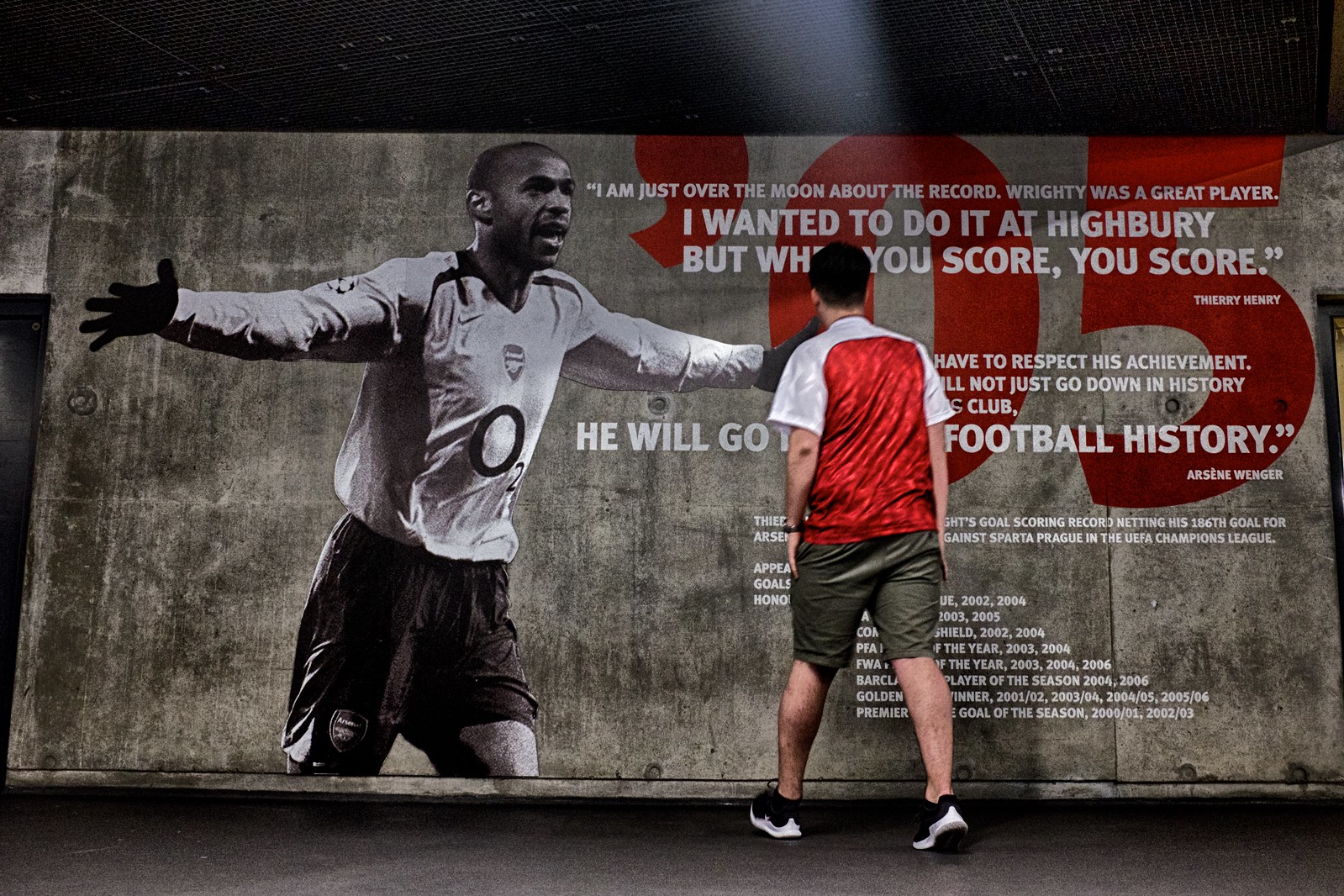In this image, a dark setting with a black ceiling, possibly a subway, is depicted. The scene is dimly lit, with a small glimmer of light illuminating a large sign. The sign features a picture of a soccer player wearing a white shirt with a large "0" (or an "O") on the front and black shorts. The image captures the player from the top half of his body down to his thighs, with his arms outstretched.

In front of this sign stands a real person, facing and looking at it. This individual is dressed in a red shirt with white shoulders, grayish-green shorts, and sneakers, and his hands are outstretched at his sides, mimicking the soccer player's pose on the sign.

The sign includes a quote attributed to Thierry Henry: "I'm just over the moon about the record. Righty was a great player, I wanted to do it at Highbury, but when you score, you score." Additionally, the sign prominently displays "05" in large red font with an apostrophe before the numbers. Part of the text seems to be obscured by the figure standing in front of it, but it appears to read something along the lines of "football history" and includes the name Arsene Wenger along with references to various years and awards.